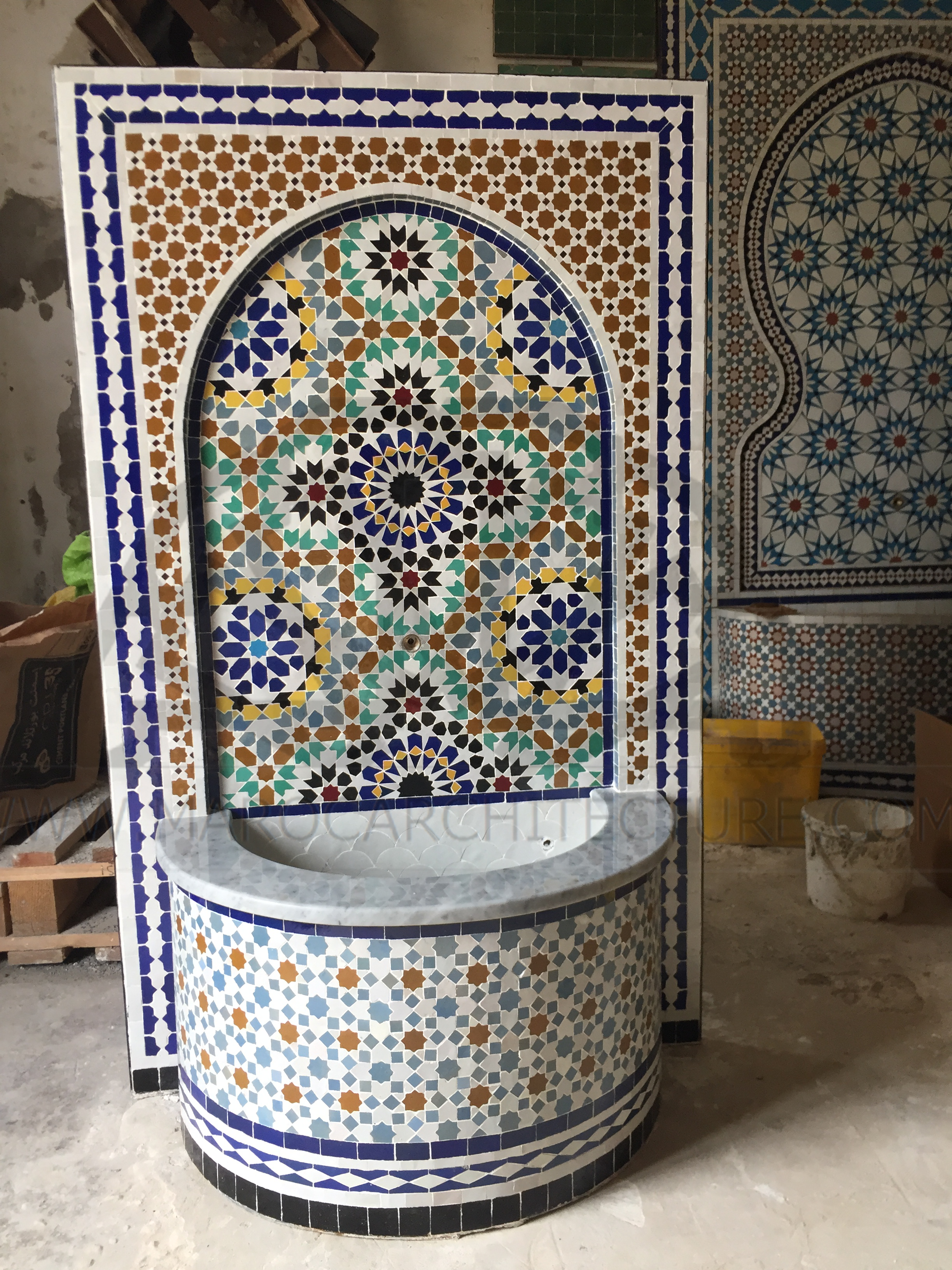The image features a large mosaic structure that closely resembles a decorative or functional piece often found in religious settings, such as a church. The central element is a cylindrical base, covered in intricate mosaic patterns with black tiles surrounding the bottom. The main design on this base consists of a white background adorned with elaborate shapes in brown and blue. This cylindrical base appears to be hollow, suggesting it might be a well or a basin of some sort.

Above the cylindrical base, there is a tall, rectangular back panel with an arched recess, which is similarly embellished with detailed mosaic work featuring small hexagons, diamonds, and stars in shades of yellow, blue, green, and black. The overall appearance and the combination of these elements give the impression of a holy water font or a small decorative fountain, reminiscent of those found in churches.

In the background, additional mosaic creations can be seen, as well as several tools and buckets—one yellow and another white, though both appear dirty—indicating an ongoing artistic endeavor or restoration process. The entire scene is set against a plain, concrete floor, adding to the workshop-like atmosphere.